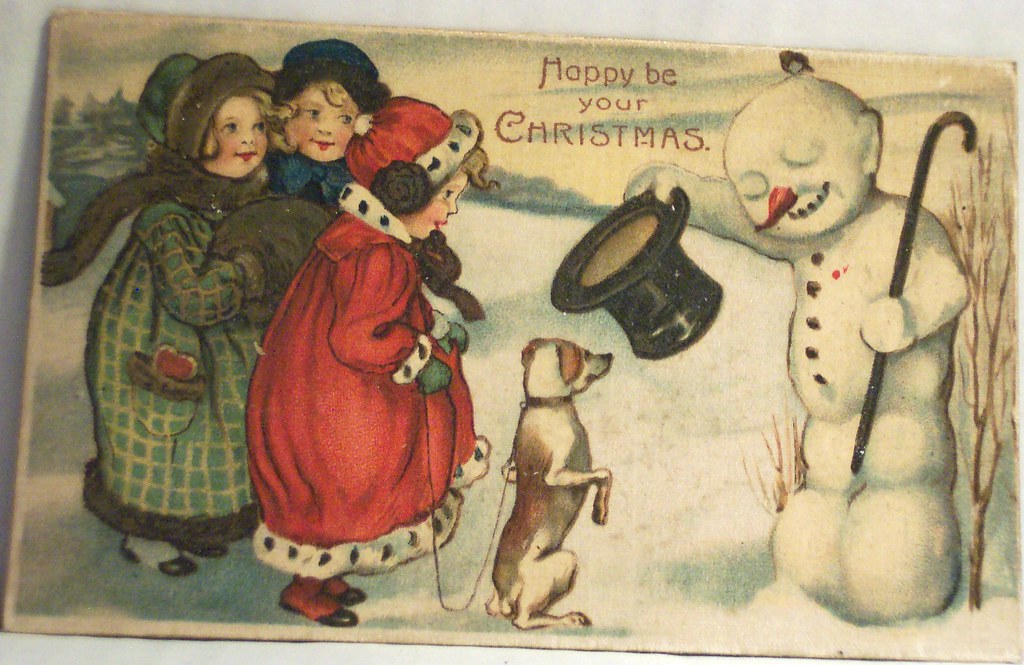The image depicts a vintage Christmas postcard, estimated to be from 80 to 90 years ago, with the greeting "Happy Be Your Christmas" prominently written in a hand-lettered red font at the top center. The card has an aged, yellowish tint, enhancing its antique appearance. On the right side of the postcard, a cheerful snowman with a top hat and black cane stands out. The snowman is detailed with coal for the mouth, a carrot nose, and eyes that appear closed, as if in greeting. The snowman holds his hat in a gesture that seems to present or greet the scene. On the lower middle left, there is a dog shown on its hind legs, seemingly begging or interacting with the three young girls positioned beside it. The girls, clad in winter clothes of various colors—red, green, and blue—stand on a snowy field. The girl in front wears a red jacket and holds a leash attached to the dog, while the two girls behind her wear green and blue jackets and hats, respectively. The card's colors include whites, blacks, grays, reds, green, a pale yellow, blonde, and beige, encapsulating the festive and nostalgic ambiance of a traditional Christmas scene.